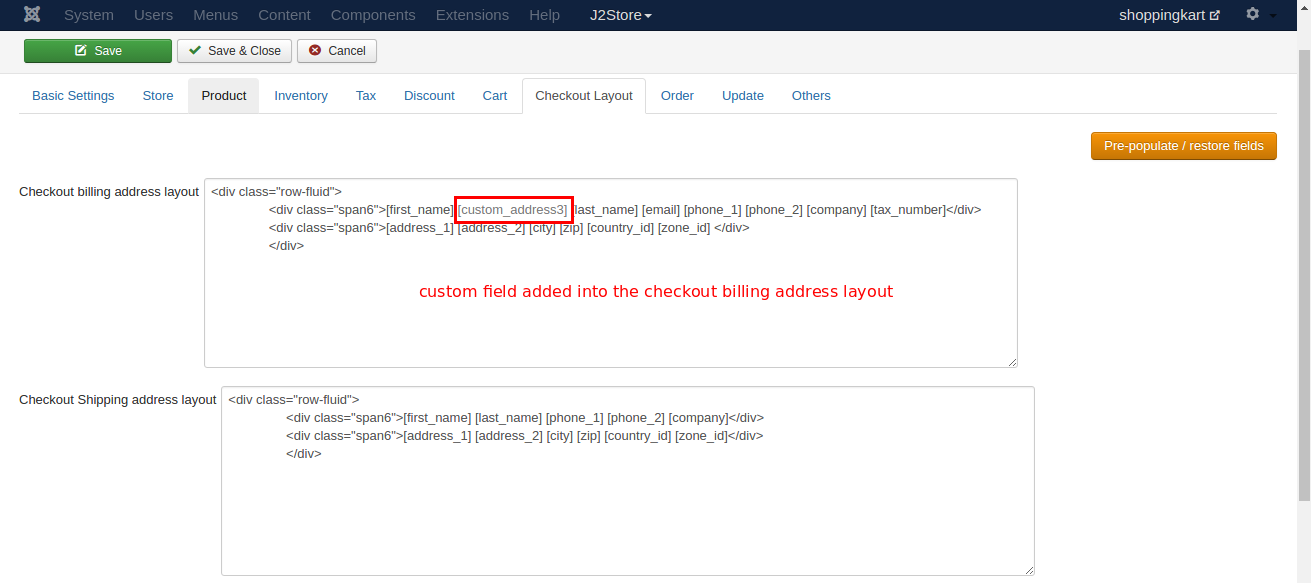Screenshot of ShoppingCart.io Website Interface

A detailed screenshot of the ShoppingCart.io website is depicted. The website’s name, “ShoppingCart.io,” is visible in the upper right corner, stylized with a “K” in place of a “C”. Adjacent to the name is a clickable button that likely redirects users to the homepage or a relevant section.

The top of the page features a thin navy blue header with multiple clickable areas. Amongst these, the “J2Store” option is highlighted, accompanied by a dropdown arrow indicating further options within this category.

The main section of the screenshot showcases a clean, white background filled with coding elements. Dominating this area are two large rectangular boxes containing lines of HTML code. The box on the left is labeled “Checkout Billing Address Layout,” suggesting that the user is in the process of designing a section of the website related to billing information.

Highlighted within the code is a section circumscribed by a red rectangle, focusing attention on the line labeled “custom_address3”. Beneath this, a red text message denotes that a custom field has been added to the “checkout billing address” layout. This detailed view indicates customization of the billing address form during the website setup process.